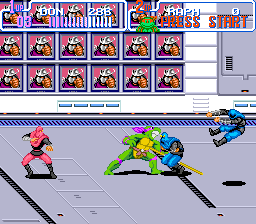The screenshot captures a moment from the classic 'Teenage Mutant Ninja Turtles: Turtles in Time' arcade game. The scene is set in a room with a gray metallic floor, featuring a blue vented strip running along the back of the room. In the background, several television monitors display images of Shredder, the iconic antagonist from the Ninja Turtles series. The floor also has distinct metallic blue and black lines.

In the center of the image stands Donatello, one of the Ninja Turtles, characterized by his green skin, yellow shell, and purple bandana. He wields his signature staff, which is extended in front of him as he engages in combat. Around Donatello are three foot soldiers: two in blue and black uniforms facing him, and one in pink and black positioned behind him. On the right side of the image runs a white strip beneath the television monitors, which includes four small blue rectangles arranged in a row. The background also features a pattern of squares framing different elements of the scene.